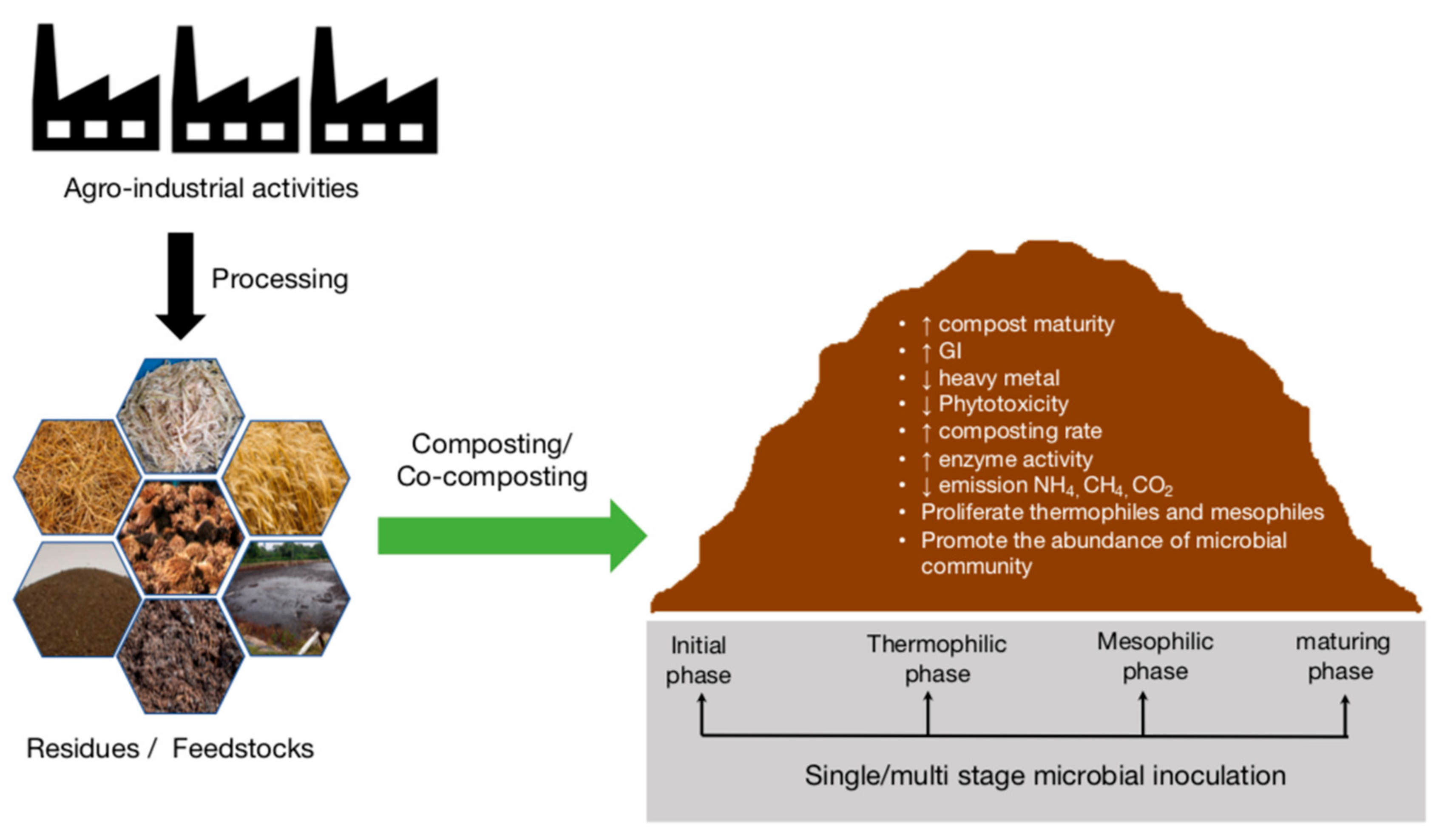This landscape-oriented diagram visually represents the composting process originating from agro-industrial activities. Starting at the top left, black-and-white illustrations of factory buildings are labeled "Agro Industrial Activities." A black arrow labeled "Processing" points downward to a cluster of seven hexagonal photographs depicting various residues and feedstocks, such as dirt, a pond, and hay. Below these images, the text reads "Residues/Feedstocks."

From here, a red arrow labeled "Composting/Co-Composting" directs attention to the right, where a graphic of a dirt mound is shown. This graphic contains white text with terms such as "Compost Maturity," "GI," "Heavy Metal," "Phytotoxicity," "Composting Rate," "Enzyme Activity," and "CO2 Emission," each accompanied by up or down arrows indicating changes or measures.

Beneath this, a gray bar charts the stages of composting with black text labels: "Initial Phase," "Thermophilic Phase," "Mesophilic Phase," and "Maturing Phase." Arrows connect these stages, illustrating the sequential process of compost development.